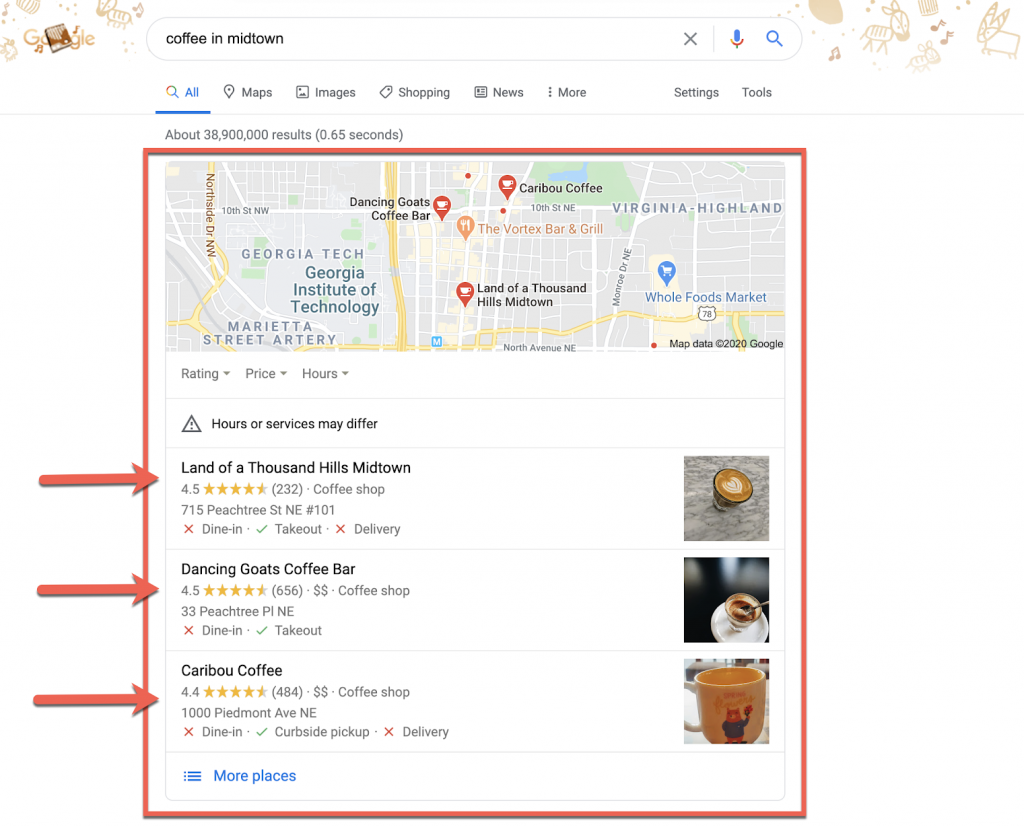The image is a screenshot from Google captured on a special themed day, likely inspired by children's drawings. The upper left and right corners feature whimsical tan-colored illustrations of zebras, horses, and music notes. Central to the screenshot is the Google search bar, which has the query "coffee in Midtown" typed in black text. Adjacent to the search bar on the right is a black "X" for clearing the text, a blue microphone icon for voice search, and a blue magnifying glass icon for initiating the search.

Directly beneath the search bar, the word "All" is highlighted in blue text and underlined. Alongside this are other searchable categories in black text such as Maps, Images, Shopping, News, with additional options under the "More" dropdown. To the right, "Settings" and "Tools" are available and clickable.

Below these tabs, the result summary indicates there are approximately 38,900,000 results found in 0.65 seconds. A red box encloses the Google search results on the left, showcasing a map of the Midtown area. The map is predominantly grey, indicating building areas, with a notable blue highlight for a small lake slightly right of center, surrounded by green parkland. A significant yellow road, indicating a highway or major road, runs left of center. The map includes labeled landmarks such as the Georgia Institute of Technology, Hilton, Land of a Thousand Hills, Midtown Caribou Coffee, and Dancing Goats Coffee Bar. 

There are three location review tags with arrows pointing to specific coffee shops. Each tag is accompanied by reviews, emphasizing user feedback. On the right side of the tags, there are Halloween-themed elements, such as glasses with spooky designs, and foam art in the shapes of ghosts and cats, suggesting the screenshot was taken around Halloween.